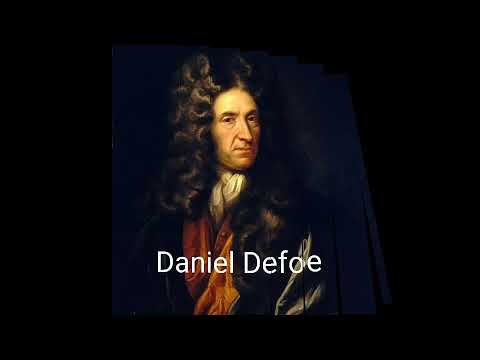This image depicts a meticulously detailed painting of a white male, presumably from the 17th or 18th century, identified as Daniel Defoe by the white text inscribed across his chest. The composition features a man with long, thick, wavy hair draping down both sides of his face, known for its deep curls and rich texture. He exudes a stern demeanor, gazing to the left. His attire includes a white scarf tied around his neck, a brown or orangish vest, and a black coat or robe overlay. The painting is framed with a black border, enhancing the historical atmosphere of the portrait.